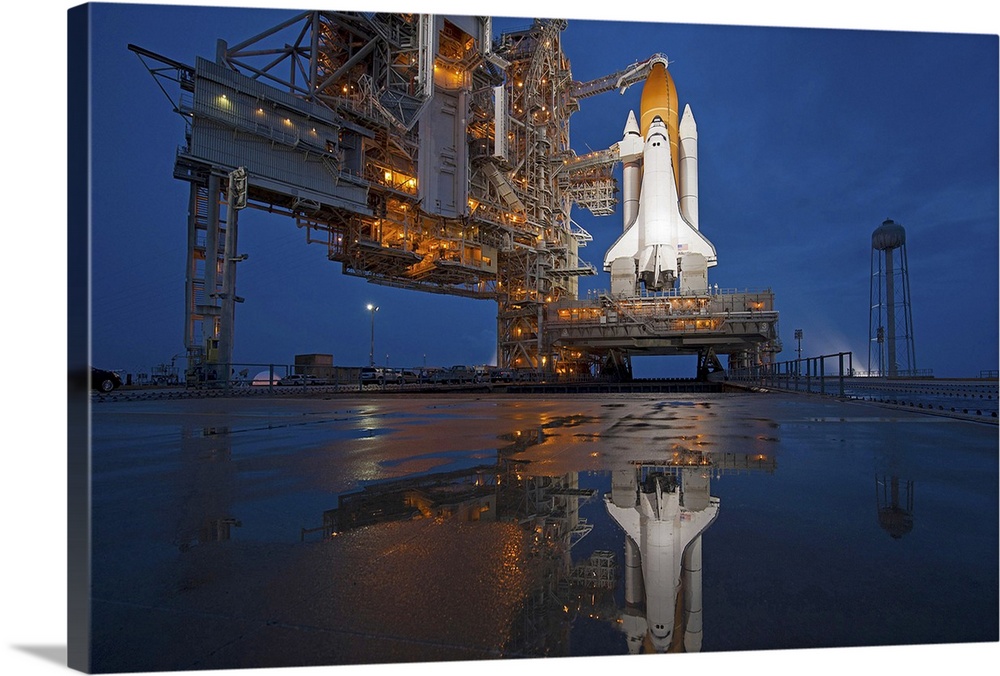In this night-time photograph, a massive Space Shuttle, its name unknown, is captured in the moments before its launch from Cape Canaveral. The image, taken from ground level, displays the imposing shuttle positioned center-right on its elaborate launching platform, which is illuminated by numerous amber lights that cast a warm glow against the dark, blue-tinged sky. The ground is wet, likely due to recent rain, and creates a clear reflection of the shuttle in a puddle below. The shuttle itself is white and prominently attached to an orange structure. To the right, there stands a tall water tower and another large structure, potentially a water retention area, adding to the complexity of the scene. The whole area is bathed in a mixture of artificial light from the launch station and the twilight hues of the sky, highlighting the anticipation and grandeur of the forthcoming launch.